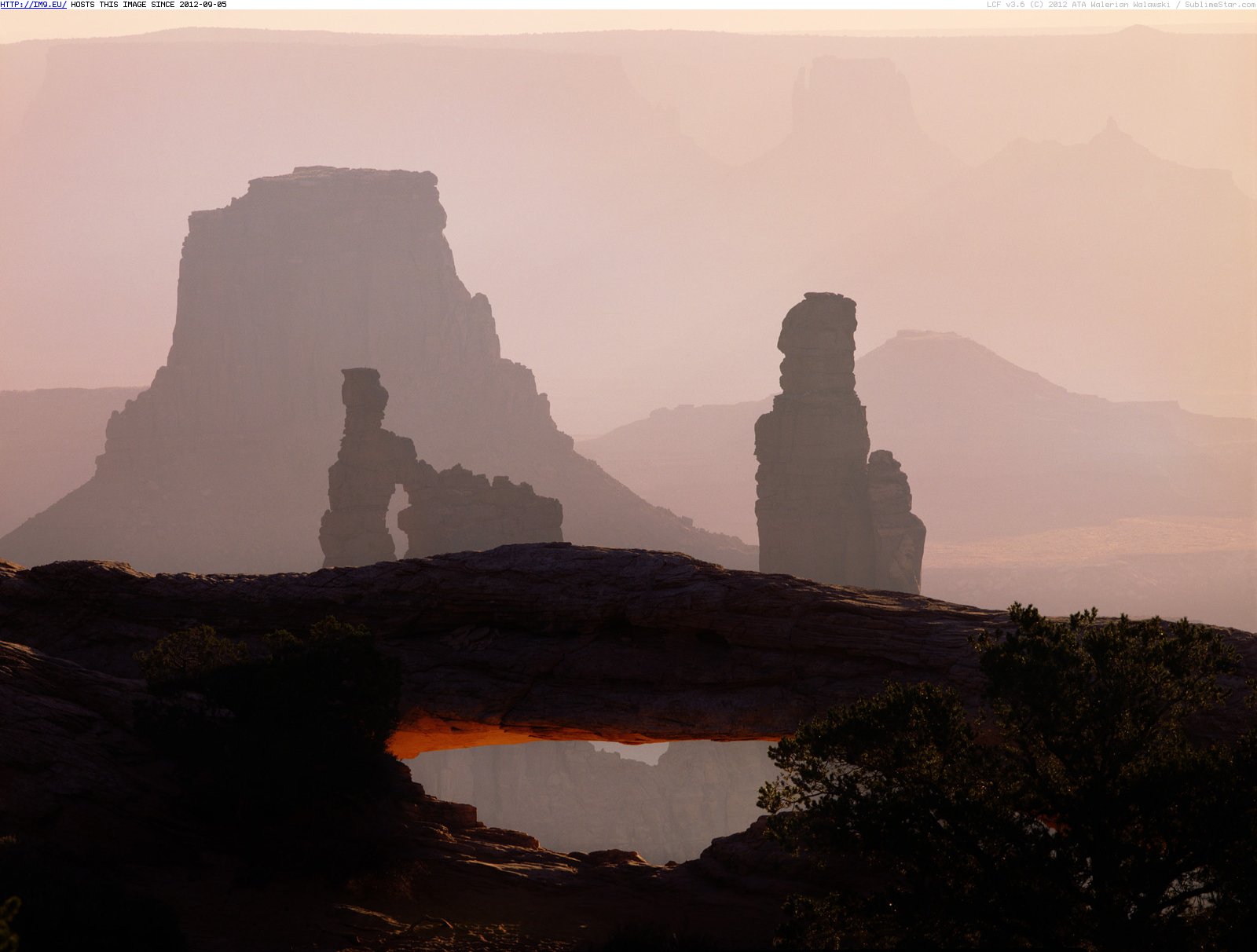In the heart of a rugged desert canyon, a striking rock formation resembling a bridge spans the frame. This natural bridge-like structure, framed by tall red and grayish-brown rocks, stands prominently in the middle of the image, with an easily walkable space beneath it. The sun casts a warm, glowing light that illuminates the underside of the bridge in a reddish hue, adding to the overall palette of grey, brown, orange, and black.

The background reveals a hazy panorama of the canyon basin, where silhouettes of plateaus and finger-like rock formations extend towards distant mountaintops, softly tinted in pink and orange hues due to dust and wind. In the bottom right corner, a surprising splash of green appears in the form of a small tree, contrasting with the otherwise arid landscape. Although tiny black text is present in the top left corner, reading "http://im9.eu" and noting that the image has been hosted since 2012-09-05, it does not detract from the natural beauty captured in this photograph. It's a cloudy day, which lends a soft, diffuse light to the scene, highlighting the textures and colors of the desert's rugged terrain.